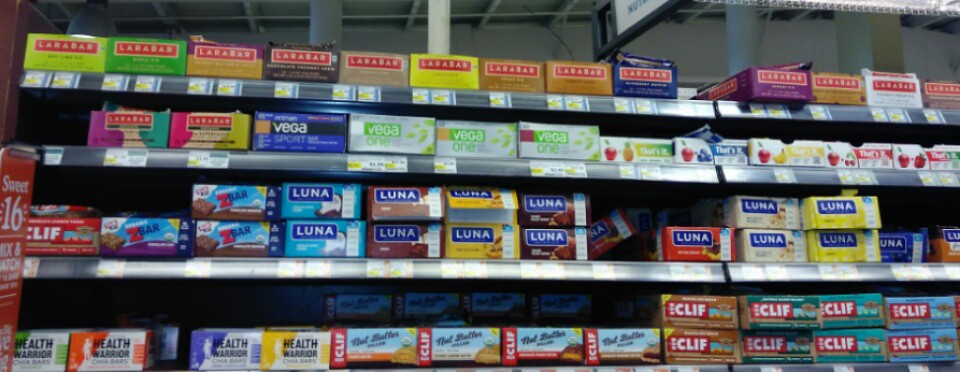The image showcases a vibrant and well-stocked grocery store aisle filled with an array of nutrition and snack bars. The scene is captured from top to bottom, with four distinct shelves of brightly colored packaged products. The top shelf is dominated by various flavors of Larabar, recognizable by their colorful yellow, green, blue, and orange boxes. The second shelf features an assortment of nutrition bars, with notable brands such as Vega and Vega One, nestled among others. The third shelf is lined with Luna bars, in a striking palette of blue, orange, yellow, and red packaging. Below these, the fourth shelf contains a mixture of Clif Bars and Health Warrior bars, in shades of green, brown, and blue. The background reveals an industrial, unfinished ceiling with visible metal pipes and parts of a fluorescent light fixture in the top right corner, adding to the warehouse-like ambiance. A partial aisle sign is located in the center of the photo, hinting at the organized and extensive selection available in this section of the store.